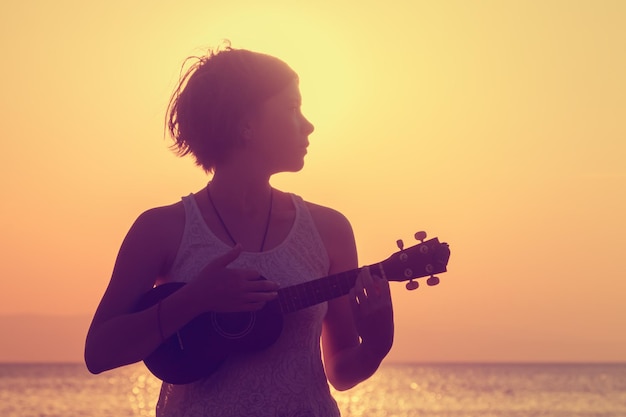The photograph captures a rectangular, horizontal color snapshot of a young girl standing at the beach during what appears to be either a sunrise or sunset, lending the scene a warm, orange-y glow. The lowest inch of the photo shows the sun glimmering on the sea, enhancing the serene coastal backdrop. The girl, likely in her 20s, has short, dark hair that falls just below her ears and is wearing a white sleeveless top paired with a dark string necklace and a bracelet on one arm. She holds a small stringed instrument, possibly a ukulele or a banjo, with her fingers positioned as if she is playing it. In the profile shot, she gazes to her left while her body faces the camera. The image is a candid snapshot, exuding a tranquil, sunlit ambiance with no text or other distractions.